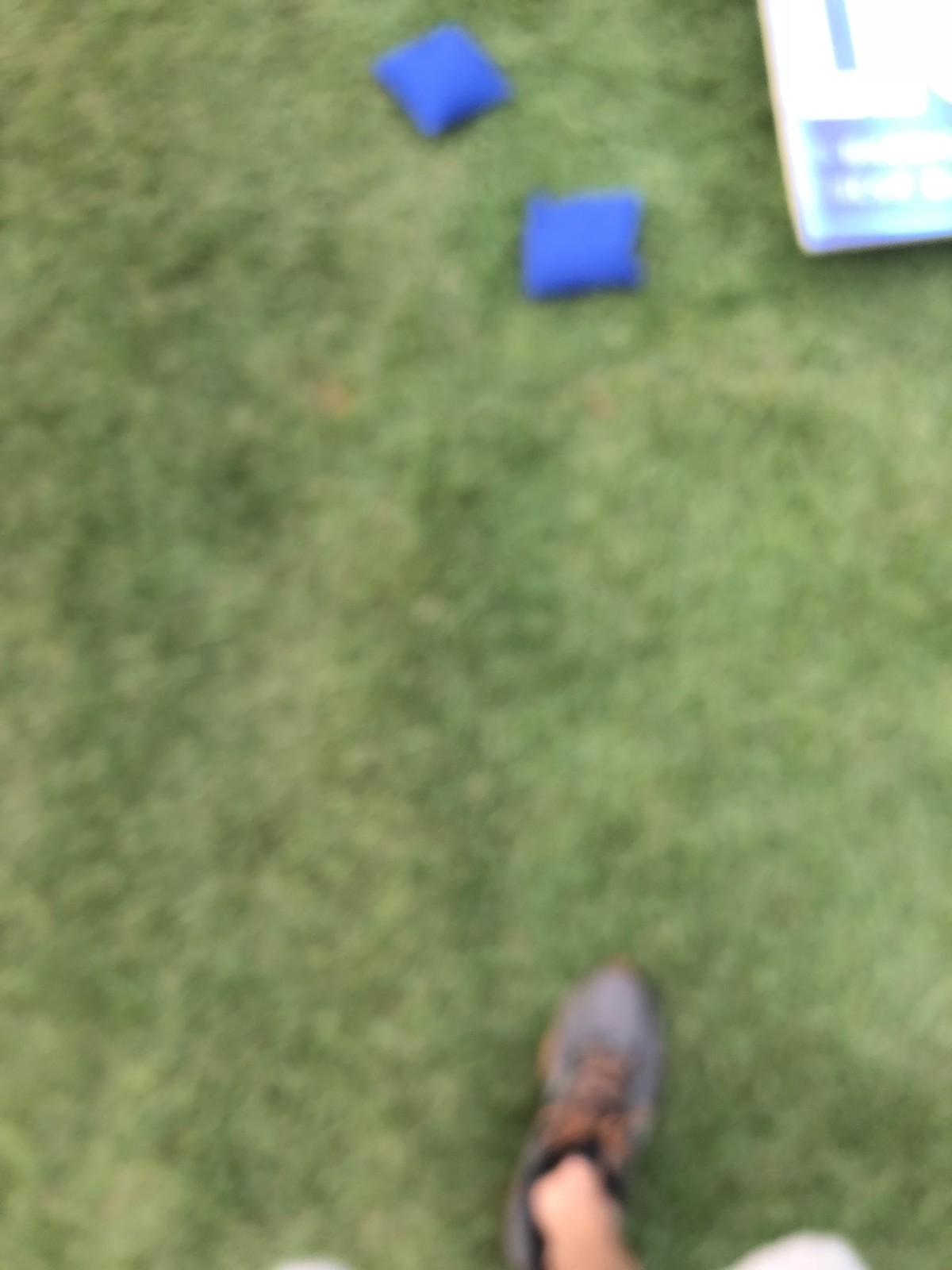In this blurry photograph, the camera seems to have struggled with focus, possibly due to lens issues or improper magnification. The picture is taken from a perspective looking straight down. Dominating the bottom part of the image is a sockless leg stepping into a brownish-orange laced gray shoe, situated on a grassy ground. The grass appears dark and light green with small splotches of brown dirt visible underneath. Towards the upper part of the photograph, there are two bright blue, square objects that resemble beanbag pillows. In the top right corner, an unidentifiable, highly reflective object catches the light, possibly a digital screen, a circus game, a board game, or merely a metallic surface. Despite the severe blurriness, the overall scene suggests a casual outdoor setting, perhaps a picnic or a park outing.